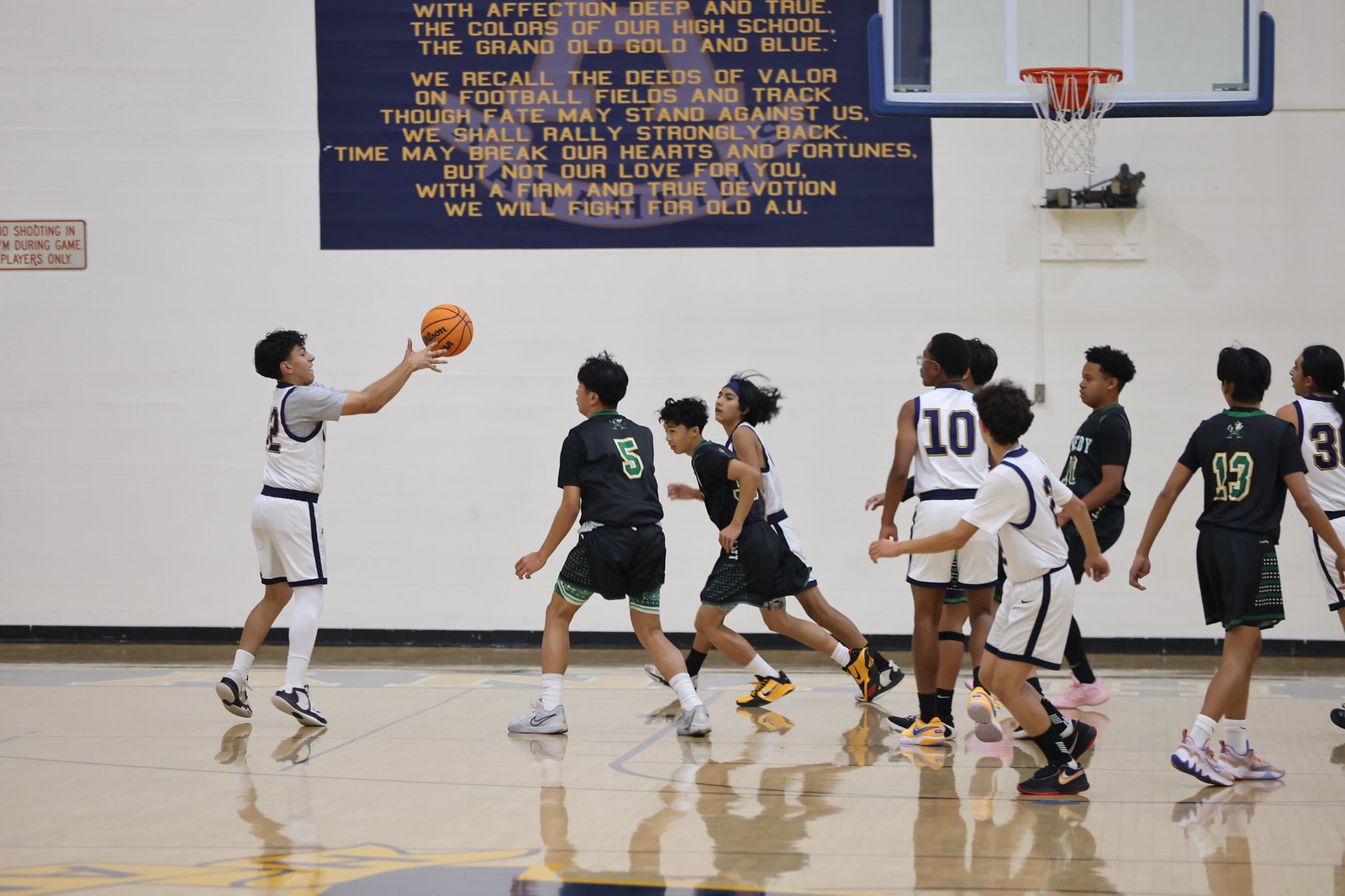The image captures an intense moment in a youth boys' basketball game set in a typical school gymnasium. The scene features nine players, likely aged between 12 to 14, actively engaged in the game. The gym has a high-gloss wooden floor and a white painted cinder block wall behind the basketball hoop, which has a see-through backboard with a blue or purple frame. Dominating the white wall is a large orange banner with gold lettering, displaying a school spirit cheer: "With affection, deep and true, the colors of our old school, the grand old gold and blue, recall the deeds of valor on football fields and track. Though fate may finally against us, we shall rally strongly back. Time may break our hearts and fortunes, but we will love for you. With a firm and true devotion, we will fight for old AU."

In the foreground, two teams can be differentiated by their uniforms. One team wears white with black trim, and the other wears black with green trim. On the left, a player in white with a ponytail and bandaged legs appears to be catching a pass, his hands raised to receive the ball that's about to enter his grasp. To his right, two players in black uniforms, one wearing number 13, are guarding another player in white. Central to the action, several players are in motion, with some obscured by others as they compete for possession. The tightly cropped photograph captures the dynamic energy of the mid-game play under the vigilant eyes of the players and the backdrop of school pride.